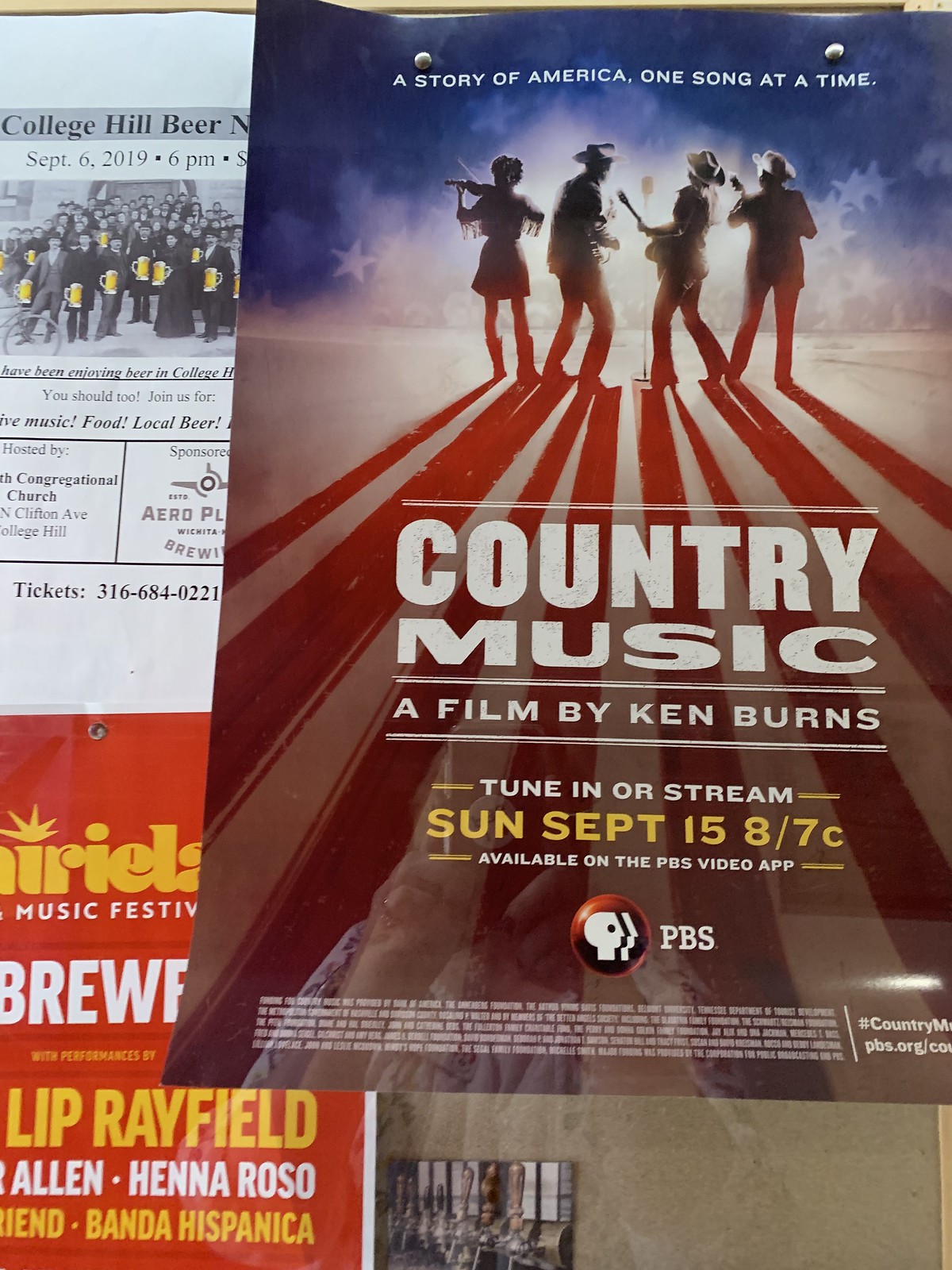The main image on this bulletin board features a prominent poster for "Country Music: A Film by Ken Burns." This poster, attached by two pins, showcases the title boldly in white letters on a red, white, and blue backdrop. At the top of the poster, it announces "A Story of America, One Song at a Time." Below, it invites viewers to tune in or stream the documentary on Sunday, September 15th at 8/7 Central, available on the PBS Video app, with the PBS logo discreetly placed underneath in a smaller, less legible font. The visual centerpiece of the poster is a group of four musicians with their backs turned toward the camera, standing on a stage. The three musicians on the right are wearing cowboy hats, while the female musician on the left, dressed in a skirt, plays a violin. Their shadows stretch towards the camera, adding depth to the scene, and a faint, translucent image of a person holding a microphone appears in the background. Adjacent to this central flyer is another partially visible advertisement for a "College Hill Beer" event on September 6th, 2019, at 6 pm, hosted by the Congressional Church on Clifton Avenue, College Hill. The flyer includes an image of people holding cartoon beers and a tagline promoting beer enjoyment in college, along with ticket information. Additionally, a red flyer for a music festival is partially obscured, its details unreadable.